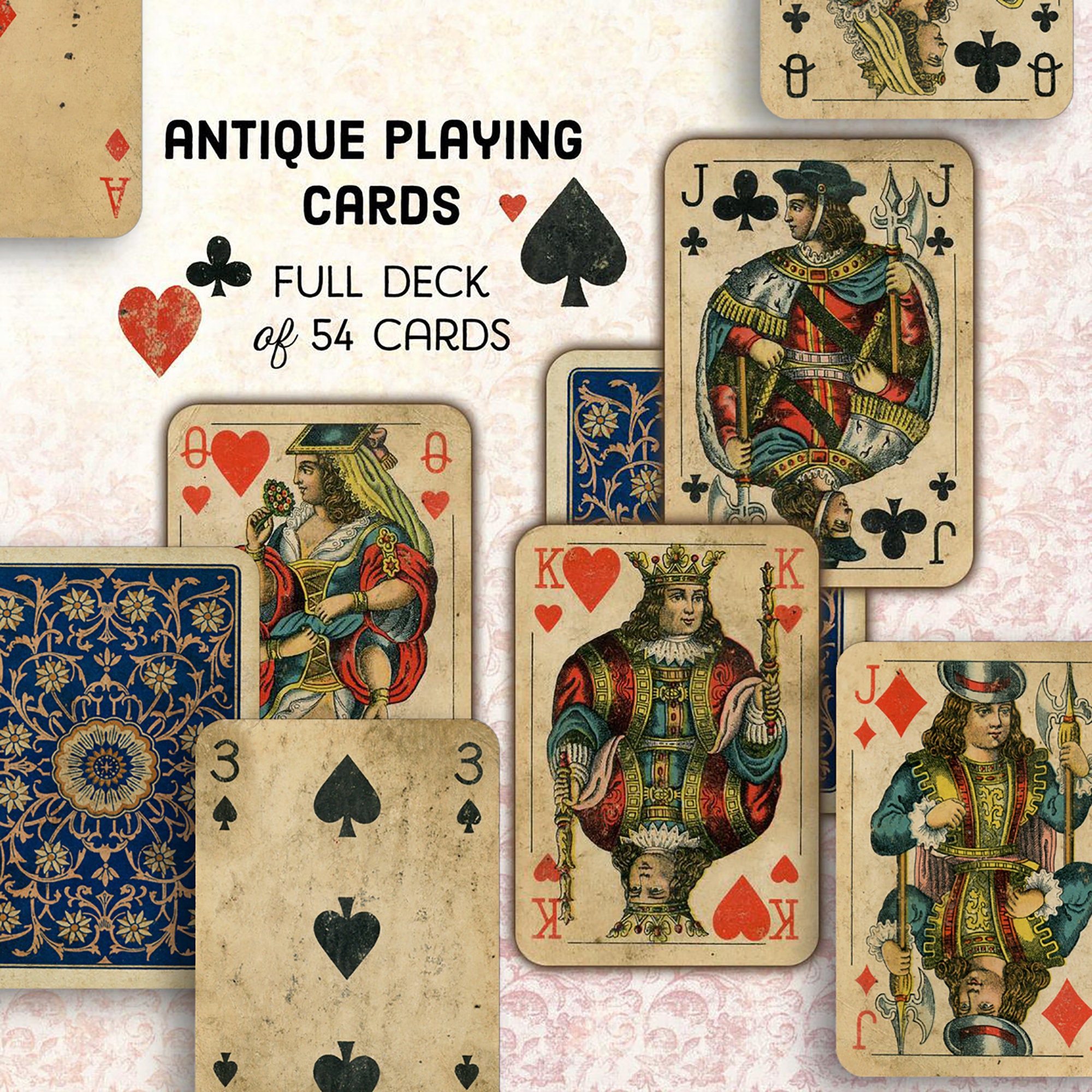The image displays a collection of antique playing cards arranged on a surface with a floral pattern on a white background. At the upper left corner, bold black text reads "Antique Playing Cards," followed by the phrase "Full deck of 54 cards" in a regular font. Accompanying the text are symbols of a heart, spade, and club. The deck includes noticeable cards such as an upside-down Ace, a visible King of Hearts, Queen of Hearts, and Jack of Diamonds, as well as a partially obscured Queen of Clubs and Jack of Clubs. Some cards are face down, revealing a blue back with floral embellishments and a white antique-looking border. The cards show signs of significant wear, displaying dirt, smudges, and a beige-and-brown taint, emphasizing their age. The overall layout appears as if intended for an advertisement, with the cards and text artistically arranged to highlight their vintage quality.